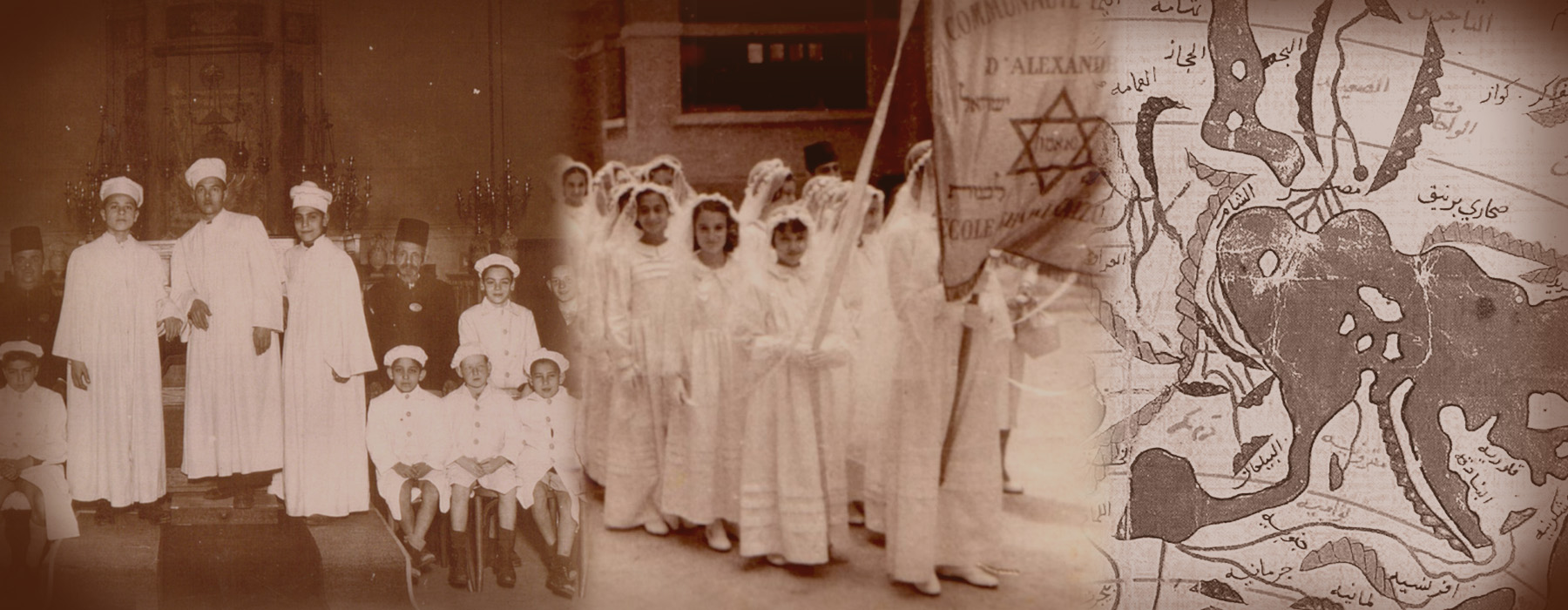The image features a complex composition divided into three separate sections, all displayed in sepia tones that give a historic feel. On the left side, three men are standing, dressed in white robes and caps, accompanied by children in shorts and white outfits with similar caps. Behind them, a man in a black hat and black robe stands. In the center, we see a group of young girls in flowing white dresses, possibly First Holy Communion attire, arranged in a formation. To the right, there is what appears to be an illustration or map, marked by brown hues, featuring a large flag adorned with a Star of David and other indistinct symbols. The background hints at a religious setting, with elements such as candles and a paned window resembling stained glass contributing to the solemn, ceremonial atmosphere.